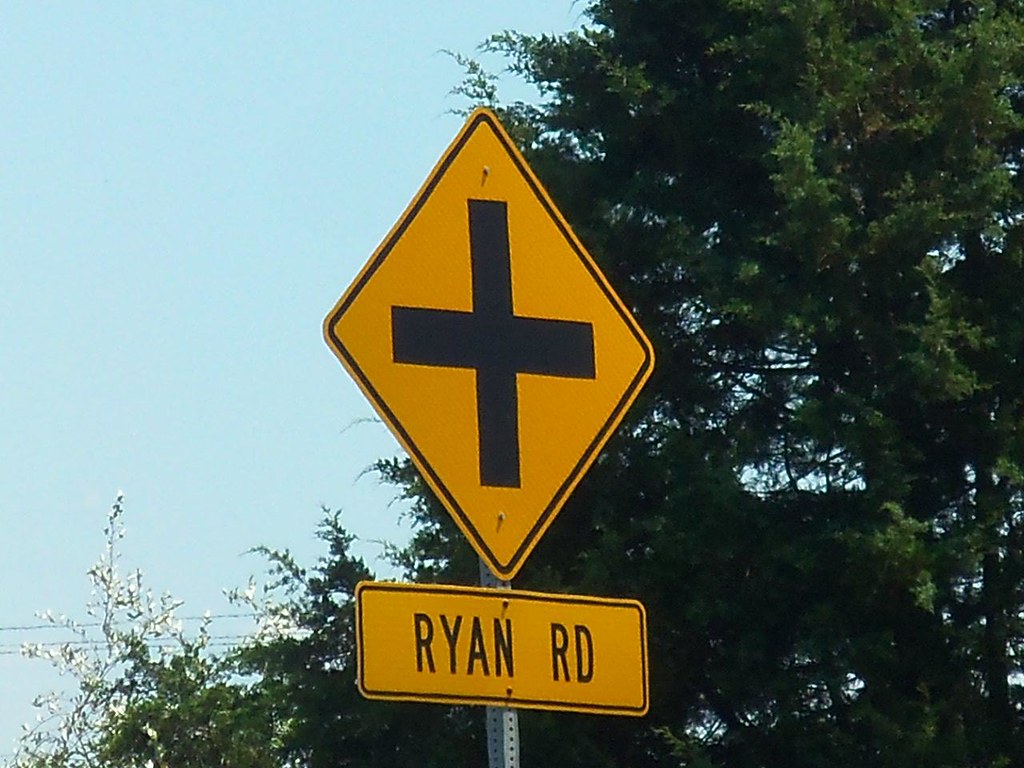In this outdoor photo, a clear blue sky serves as the backdrop, accentuated by a collection of trees that progressively increase in height from left to right. Positioned centrally is a metal pole with numerous drilled holes visible along its length. Attached to this pole are two signs: the top is a yellow diamond-shaped road sign outlined in black featuring a thick black cross, indicative of an intersection. Below it, a rectangular yellow sign displays the words "Ryan Road" in bold black letters. The scene depicts the lush greenery of the trees, suggesting a summertime setting, and a faint glimpse of a telephone wire pole amidst the foliage.